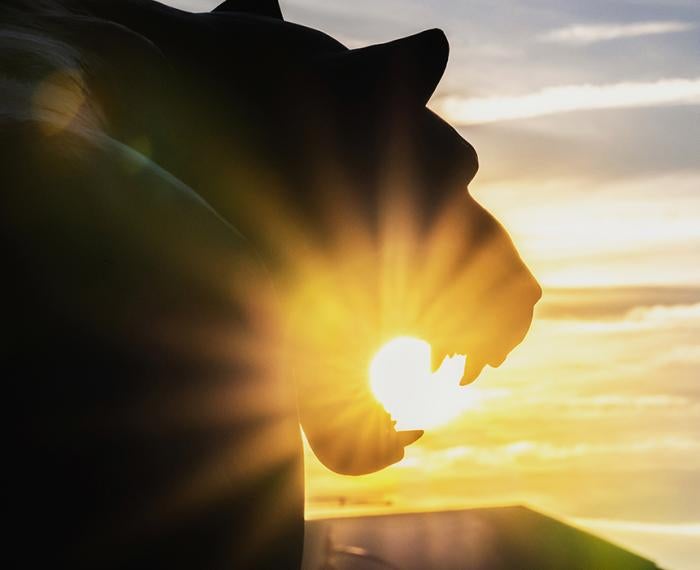The image is a striking photo capturing the side silhouette of a tiger statue during a close-to-sunset moment. The tiger's distinct features, like its ears, eyes, nose, and open mouth showcasing its sharp teeth, are beautifully outlined against a vividly transitioning sky. The sky presents a gradient of blue at the top and orange-yellow near the horizon, accented by stripes of clouds. In the centerpiece of the photo, the setting sun is perfectly positioned within the open mouth of the tiger, emitting intense rays of sunlight that illuminate the statue’s silhouette and create a dazzling spectacle of light. The photo, formatted in a square rectangle, vividly captures the glowing sunlight streaming through the statue's mouth, highlighting the powerful contrast between the dark form of the tiger and the radiant sky.